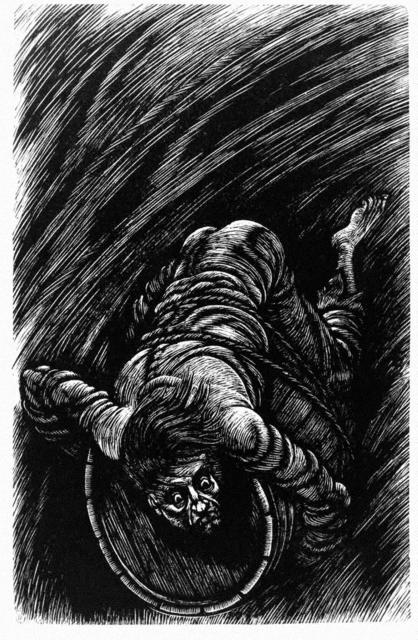In a striking black and white lithograph evoking a deeply nightmarish mood, a malnourished and horrified man is depicted lashed with rope to a wooden barrel adrift in tumultuous waters. Barefoot and with long, disheveled black hair, he clings to the barrel in a desperate bid for survival. His terrified gaze meets the viewer, his face oriented towards the bottom of the image while his legs and rear end are seen lifted towards the top, revealing the ropes binding him. The shading is dense and dark, contributing to the morbid atmosphere, and creating an impression of immense struggle and despair in the stormy seas. The man's pained expression and vulnerable posture evoke a heavy emotional response, making this etching a haunting visual narrative of extreme distress and helplessness.